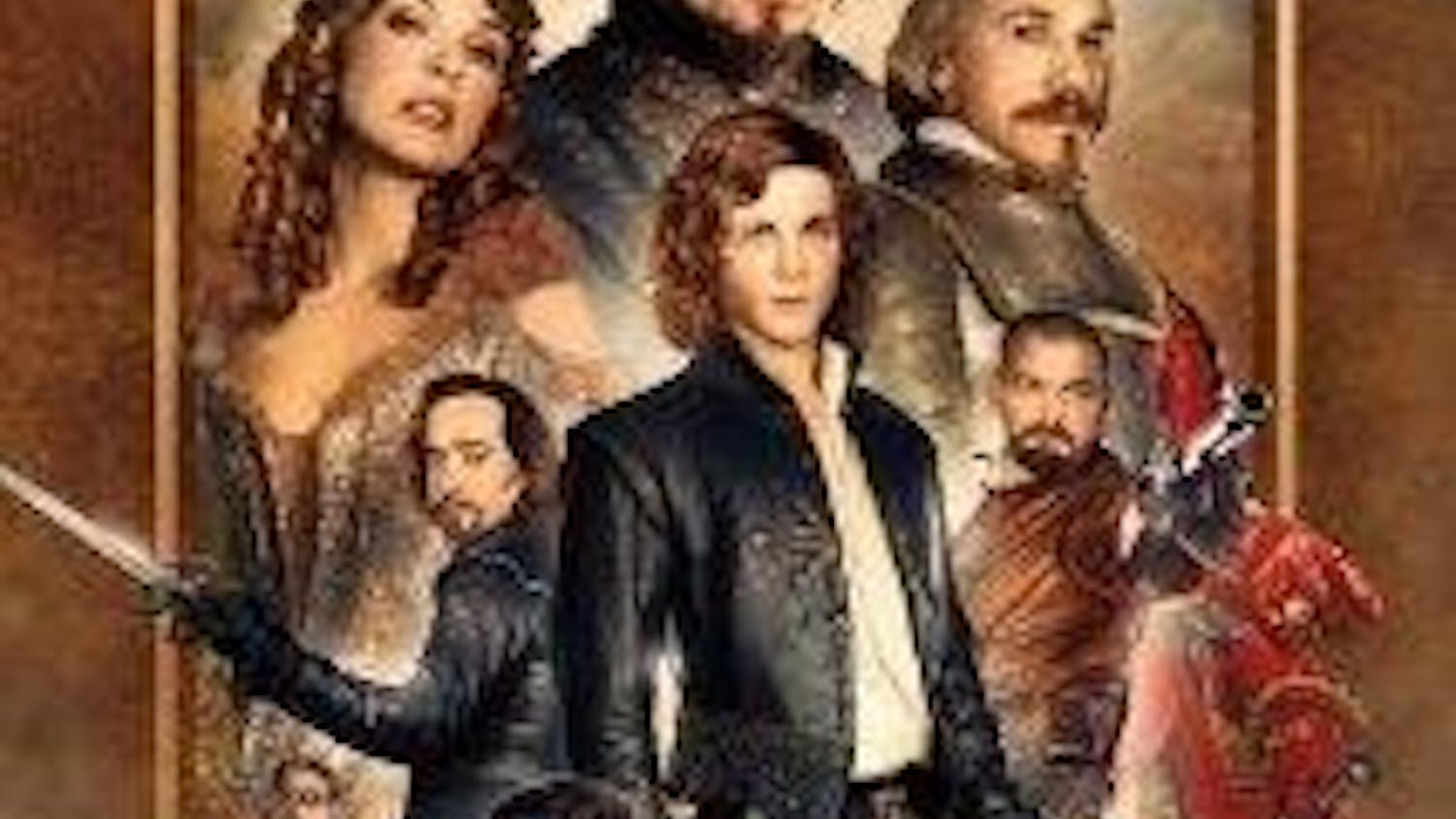This image appears to be an advertisement for the mid or late 2000s movie "The Three Musketeers," featuring characters in detailed period attire reminiscent of the 17th or early 18th century. Despite its very pixelated, low-resolution quality, some details can be discerned. In the center foreground is a young man with long brown hair, dressed in a cutaway jacket with a white shirt underneath. He has a prominent role, as indicated by his foreground placement. To his left is a man with a shaved head and a brown beard, holding a musket and dressed in a rust-colored vest. Another character to the young man's right is seen holding a sword and wearing a black leather jacket, sporting a black goatee. Above these figures, a woman with long curls and a low-cut bodice adorned with brown ruffles stands to the left, while an older man, possibly Christoph Waltz, is on the right, dressed entirely in black clothing. This composition includes six characters, all in period attire, arranged in a way that suggests a powerful, dramatic narrative fitting of a movie poster.